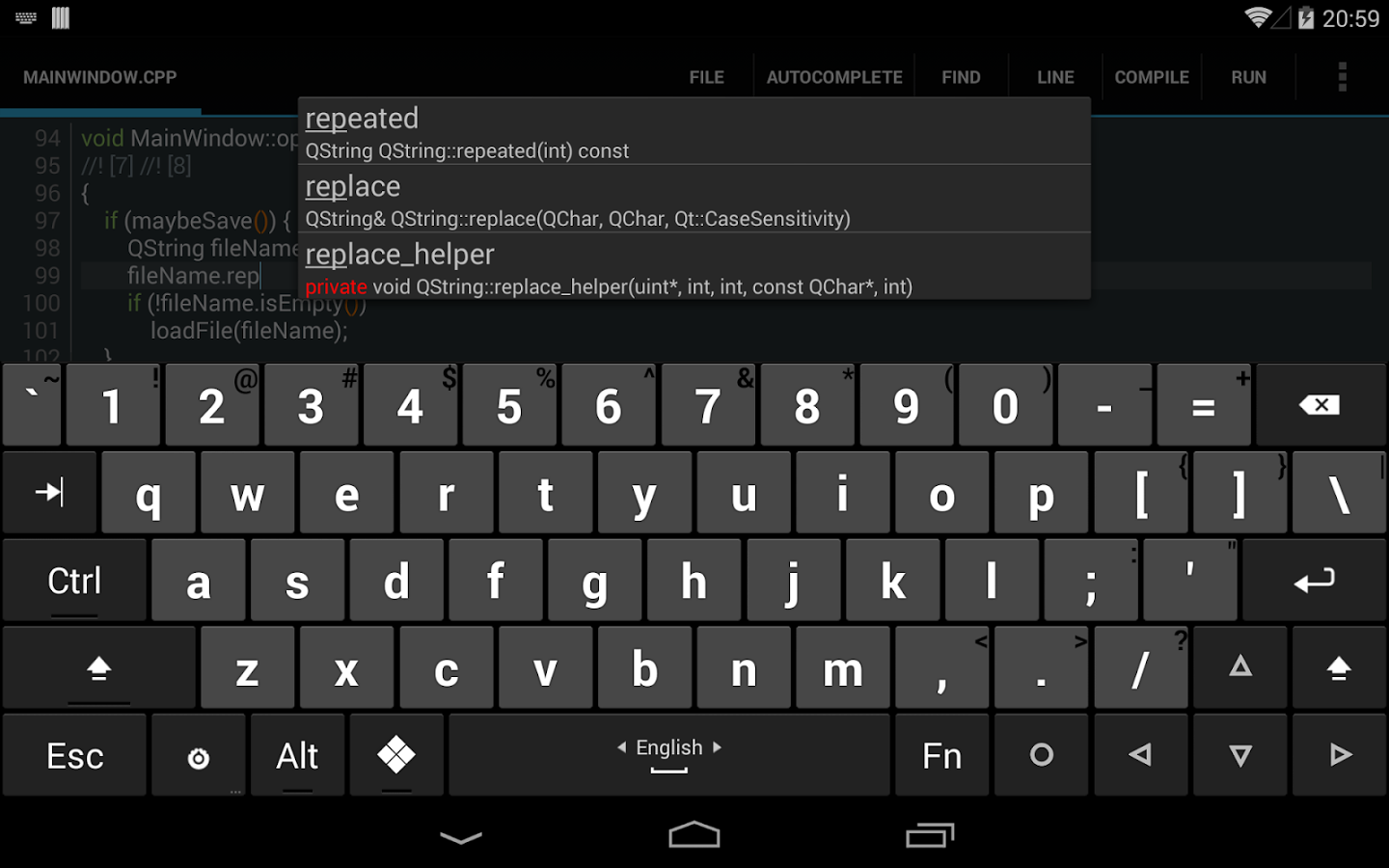A detailed screen capture of a coding environment on a desktop interface is displayed. The background is predominantly black with contrasting grey and white text. At the top of the screen, there are various icons including a keyboard and a piece of paper symbol. Moving towards the right, other icons like a Wi-Fi signal indicator, a battery level icon, and the digital time reading "20:59" are visible.

In the main section of the screen, a window titled "mainwindow.cpp" is open. The interface shows menu options such as File, Autocomplete, Find, Line, Compile, and Run, followed by an ellipsis. The window appears to be actively locating some files, with visible lines numbered from 94 to 102. Keywords like "void" in green and operational requests are present in the code snippet.

A blue progress bar is situated near the top of the interface, partially obscured by a grey dialogue box with white text. This dialogue displays coding terminology including "Qstring," "repeated," "int const," "replace," "Qchar," and "QT case sensitivity," along with function names like "replace_helper" highlighted in red and other private functions and parameters.

At the bottom section of the image, a virtual keyboard is displayed, characterized by shades of grey with white key labels. Additionally, a row of icons is present, featuring a down arrow, a house symbol, and an icon depicting two overlapping squares, providing quick navigation options.